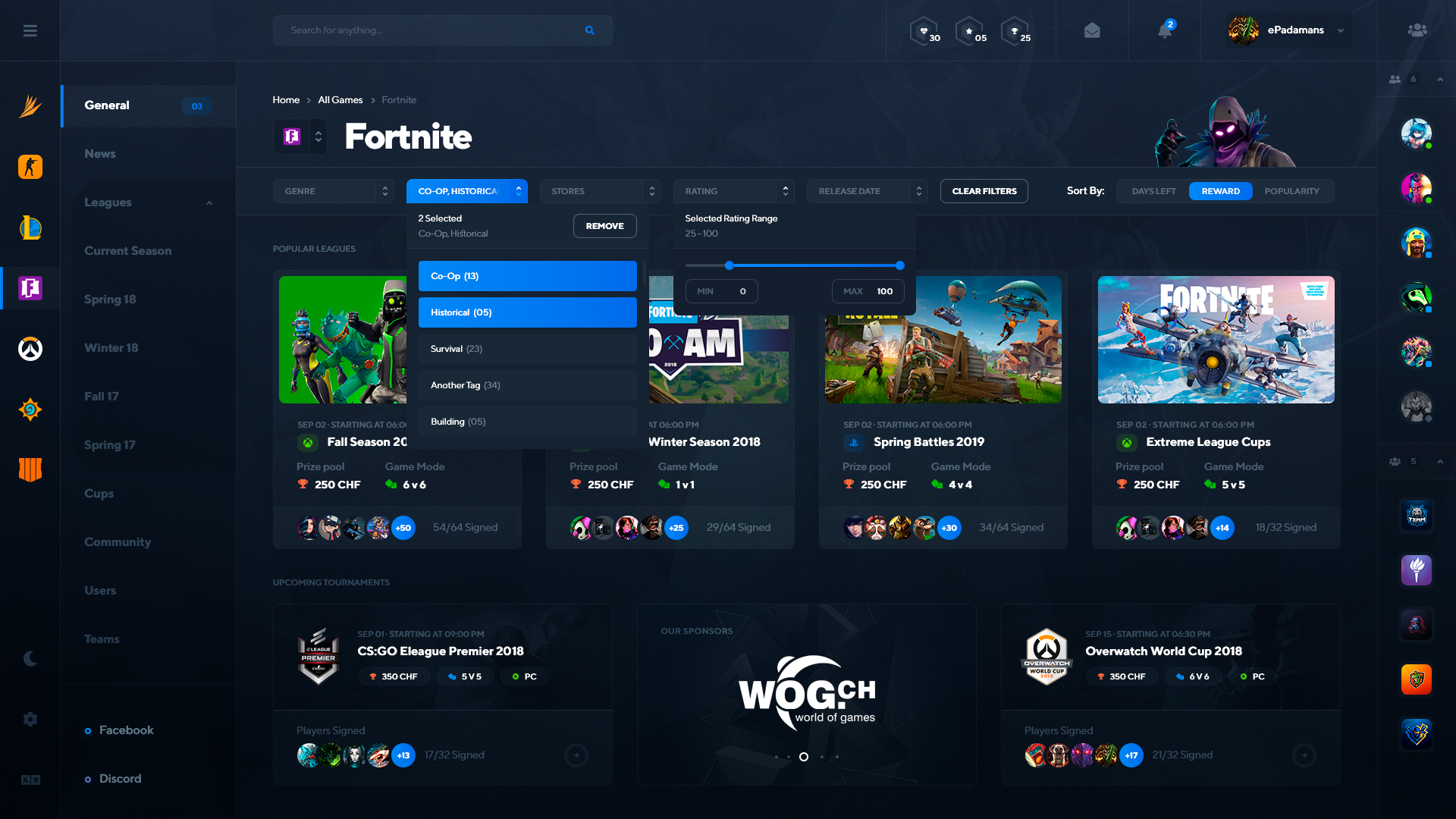The image depicts a gaming website or interface from a gaming application, characterized by its dark gray, textured background. On the left side, there is a vertical navigation menu with various clickable tabs. These tabs include categories such as "General News," "Leaks," and seasonal labels like "Spring 17," "Fall 17," and "Winter 17," among others. Near the bottom of this menu, logos for Facebook and Discord are visible.

At the top left corner of the interface, there is a search bar, while the top right corner features various icons including the user's profile picture and profile name. The screen is currently focused on the "General" tab, prominently displaying the word "Fortnite" in bold white letters. Below this heading, there are additional sub-tabs and several images, likely showcasing gameplay results and highlights from Fortnite.

On the right side of the interface, there is a column featuring profile pictures of the user's online friends.